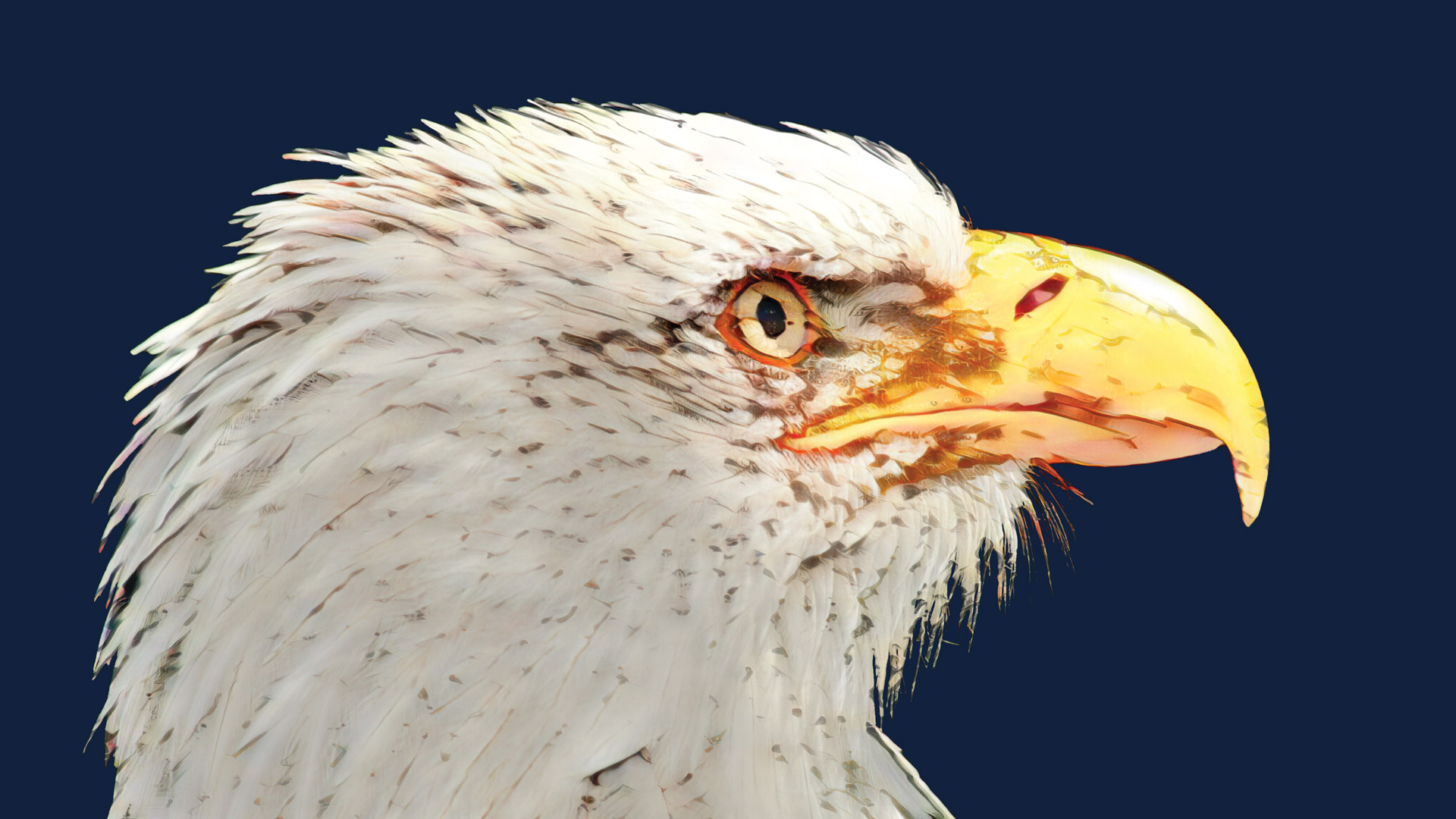This close-up image features the head of a majestic bald eagle, captured in a photograph against a solid royal blue backdrop that paradoxically resembles a painted canvas. The bird, seen from its neck to the top of its head, boasts a plume of white feathers that lay flat against its face. The feathers are pristine white, interspersed with subtle brown markings and dots. The eagle's striking yellow beak, which curves sharply at the end, has a red nostril mark and shows signs of wear with visible scratches. Only the bird's right eye, bright and open with an orange ring around it and an iris that seems almost as white as its feathers, is visible in this detailed portrait.